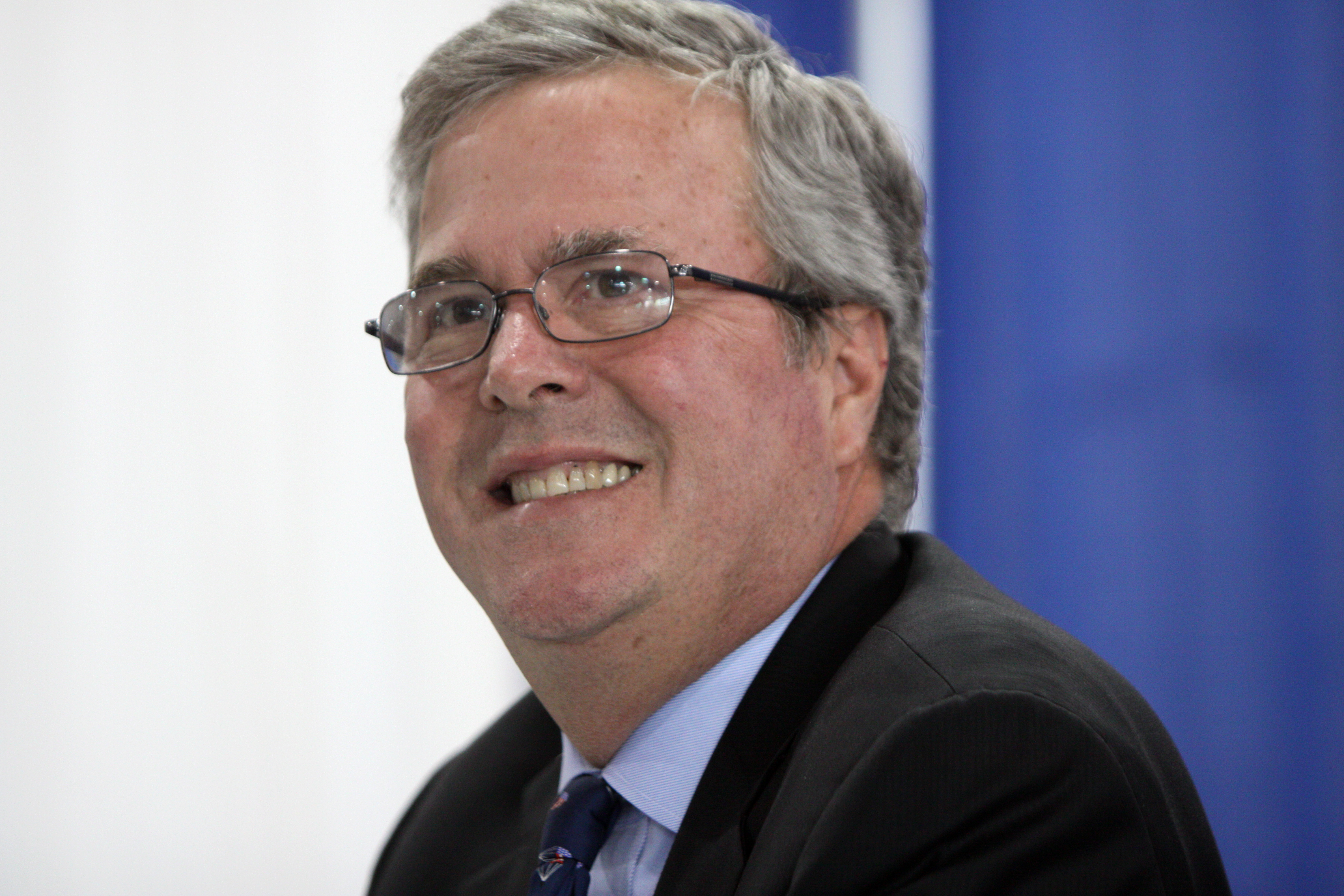This photograph captures Jeb Bush, a white man in his 50s or 60s, wearing glasses and a business suit. His short hair is a mix of gray and black. He sports an awkward grin, displaying tall teeth that appear slightly yellow. He is dressed in a dark-colored suit jacket, a light blue dress shirt, and a dark blue tie. The background of the image is a mix of dark blue and light blue, with a distinct vertical white mark above his head. Jeb is positioned slightly to the left side of the image, appearing to look out of the left corner of his eye towards something or someone off-camera. The setting looks to be indoors with a somewhat blurrier backdrop, adding focus to his facial expression and attire.